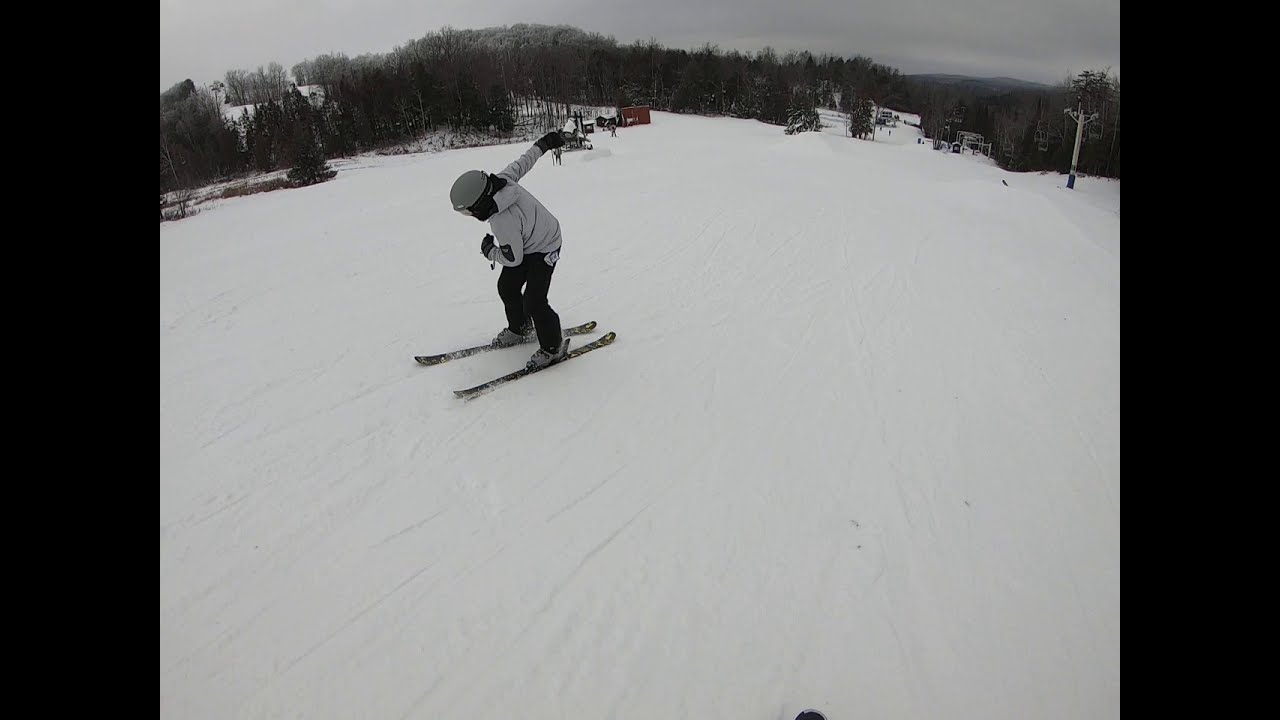In this striking winter scene, a skier clad in a grey helmet, grey jacket, and black ski pants fiercely glides down a pristine, fresh-snow-covered hill, surrounded by a crisp and chilly atmosphere indicated by the overcast, grey skies. The skier, exhibiting dynamic motion with arms slightly behind and to the sides, propels down without ski poles, possibly in practice or warming up. Tracks from previous skiers crisscross the snow, adding texture to the landscape. The background showcases a serene line of brown trees dotting the snowy landscape, a ski lift, and small shacks or cabins, including a distant red cabin, giving the scene depth and context. The overall ambiance is somber and cold, amplified by the dense clouds overhead, encapsulating the quintessential vibe of a grey, snowy day at a ski resort.